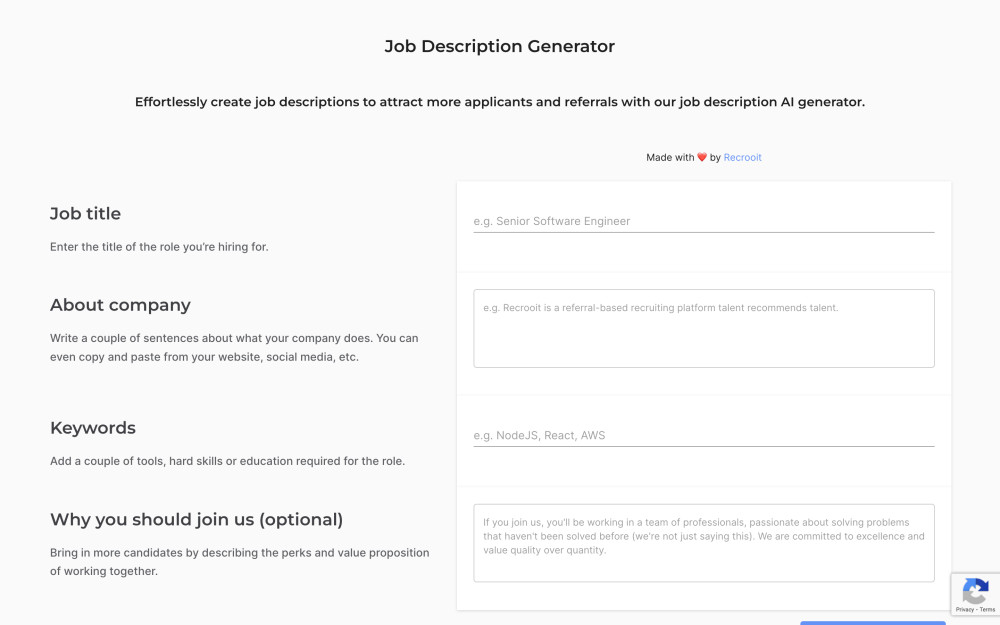This screenshot captures a desktop interface of an AI text generator program, designed for creating detailed job descriptions. The interface features a primarily gray background with black and gray text. 

At the top of the screen, black text reads "Job Description Generator," followed by a subheading: "Effortlessly create job descriptions to attract more applicants and referrals with our job description AI generator." 

On the left-hand side, four different input categories are visible, each accompanied by their respective descriptions:
1. **Job Title**: Users are prompted to enter the title of the role they are hiring for. Next to this prompt, a white input box with gray placeholder text reads "e.g. Senior Software Engineer."
2. **About Company**: This section instructs users to write a couple of sentences about their company, suggesting they can copy and paste text from their website or social media. Adjacent to this, a white input box bears gray placeholder text suggesting examples.
3. **Keywords**: Here, users are asked to add tools, hard skills, or educational requirements for the role.
4. **Why You Should Join Us (Optional)**: This final section encourages users to bring in more candidates by describing the perks and value proposition of the role, enhancing the attractiveness of the listing.

The UI elements are clearly laid out, guiding the user through the process of creating a comprehensive job description with the aid of AI.